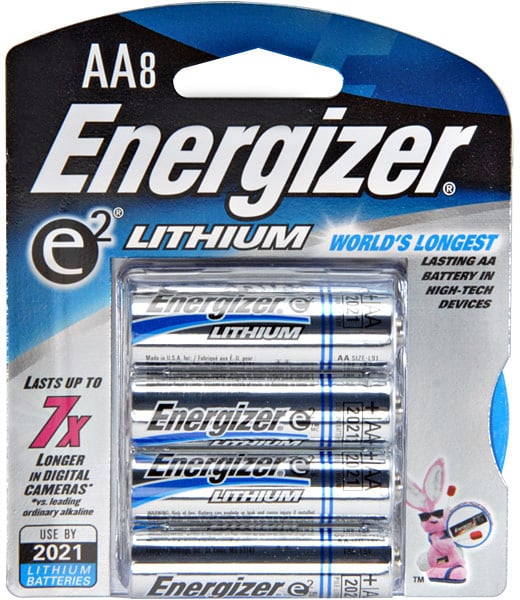This image depicts a package of Energizer AA lithium batteries. The packaging is primarily composed of a cardboard material, featuring straight sides and a rounded top with a hole in the center for hanging. The top right corner is blue, and the color transitions to black down the middle. The main area at the bottom of the package is gray.

In the upper left corner, large white letters "AA" and the number "8" are prominently displayed, indicating the battery size and quantity. Directly beneath this, the brand name "Energizer" is written in bold white letters across the midsection of the package. To the right of the brand name, there's a distinctive circle with a lowercase "e" and a number "2" beside it.

Beneath the circle, the word "lithium" is written in white, followed by the phrase "world's longest" in blue. Below this, in black text, it states "lasting AA battery for high-tech devices." A transparent plastic rectangle runs vertically down the center of the package, through which rows of gray batteries with a blue stripe and the inscription "Energizer lithium" can be seen.

In the bottom left corner, the text "lasts up to seven times longer in digital cameras" is displayed, with "seven times" highlighted in red. Below this statement, a small square notes the expiration date, "used by 2021." The phrase "lithium batteries" appears in blue text adjacent to this square.

Finally, in the bottom right corner, there is an image of the iconic Energizer pink bunny, wearing black sunglasses and carrying a drum.